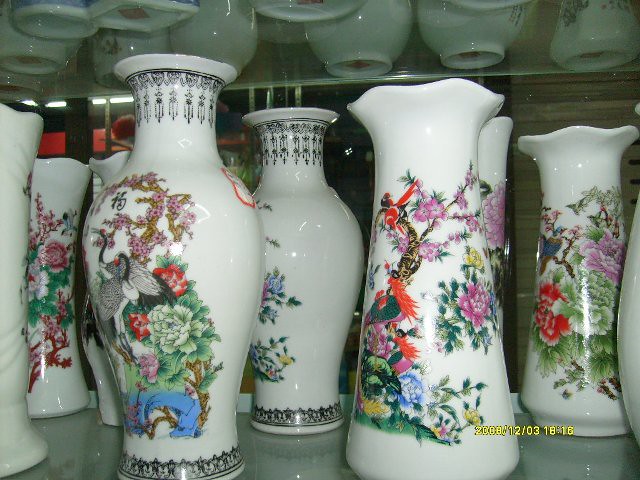This photograph, dated December 3, 2008, showcases a collection of intricately designed oriental vases, likely of Chinese or Japanese origin, displayed inside a glass case at eye level. There are eight vases visible, arranged in a pattern with at least two rows. Despite some being partially obscured, three vases can be seen in detail. Each vase is predominantly white and adorned with colorful floral patterns and depictions of birds, including cranes and other feathery species. While some vases have elaborate black borders and scrollwork at the top and bottom, resembling dangling earrings, others feature a plain fluted top. The vases vary in shape, with some having open tops showcasing vibrant colors such as pink, red, blue, and green. The designs share a thematic family resemblance, suggesting they might be variations of the same illustration.